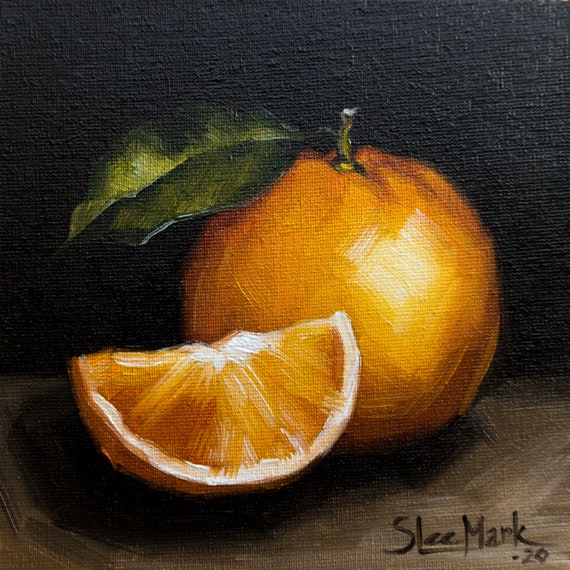This is an oil painting on canvas that showcases a vivid depiction of an orange. The composition features a whole orange positioned centrally, boasting a vibrant orange hue and a short stem with a dark green leaf extending to the left. In front of this, towards the lower left corner, lies a fresh orange slice, displaying the juicy segments and contrasting white pith. The entire setup is set against a striking black background, with the fruits resting on a grayish-brown surface. The artist's signature, "S. Lee Mark - '20," is elegantly placed in the lower right-hand corner of the painting, lending authenticity to this beautifully detailed art piece.